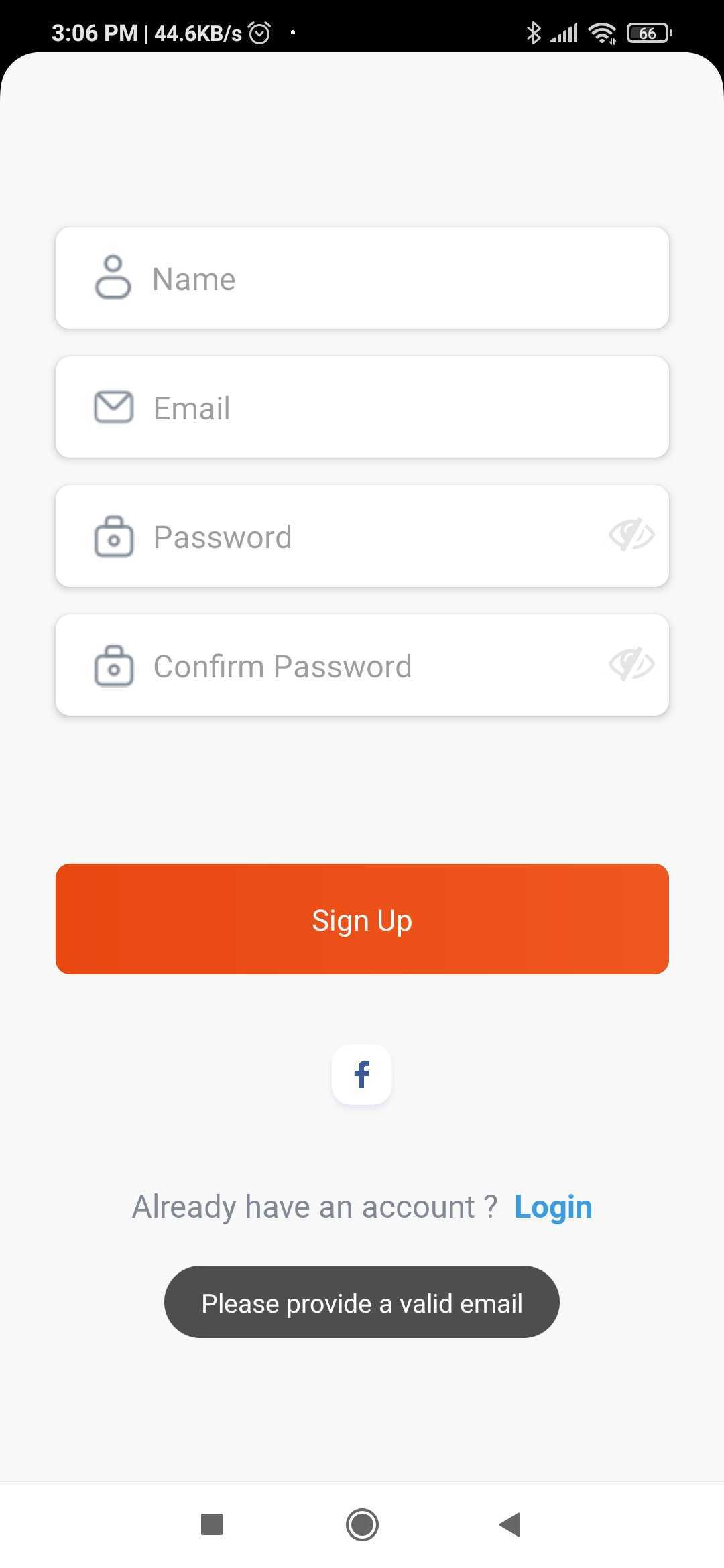A detailed screenshot from a smartphone interface at 3:06 PM. The status bar at the top shows a data transfer rate of 44.6 kbps, accompanied by a clock icon and a dot. To the right, there are icons indicating active Bluetooth, full cell signal, full Wi-Fi signal, and a battery at 66%. 

In the central light gray section of the interface, four input fields are displayed. The first field shows a silhouette icon labeled "Name," the second field features an envelope icon labeled "Email." The third and fourth fields, both illustrated with briefcase or lock icons, are labeled "Password" and "Confirm Password" respectively. Each of these two last fields includes an icon of an eyeball with a line through it indicating the obscured visibility of the typed passwords.

Below these fields, there is an orange button with slight rounded corners, featuring bold white text that reads "Sign Up." Further down, there is a white square with rounded corners containing a dark blue "F," symbolizing Facebook. Underneath, a message in gray text reads "Already have an account?" followed by a hyperlinked blue text "Log In." At the bottom, a black oval button with white text displays the message "Please provide a valid email."